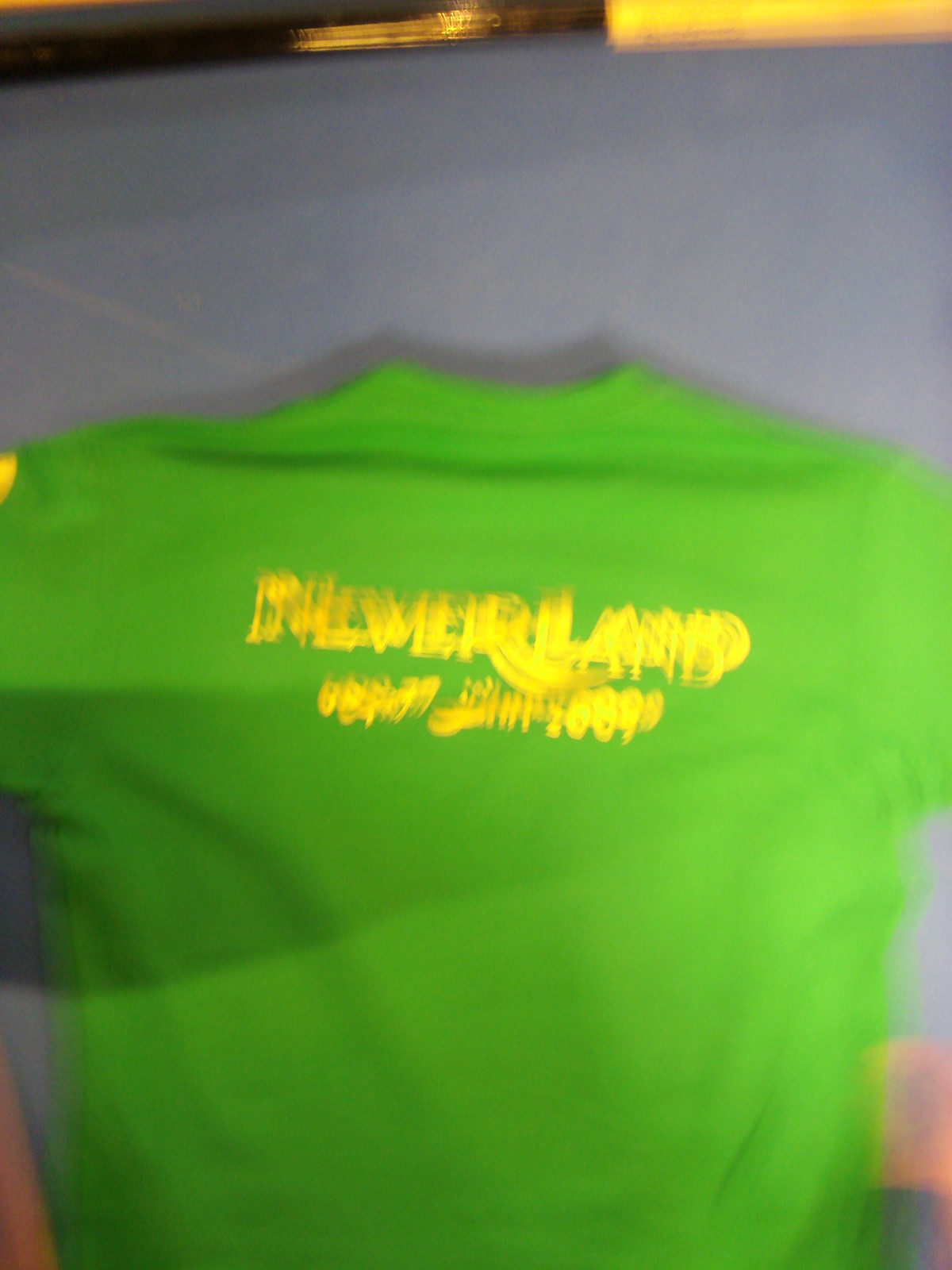The image features the back view of a green athletic jersey. Prominently displayed on the upper part of the jersey are large, bright yellow letters and numbers, which appear to spell out a name—likely "Powerland." The text is slightly obscured, making it difficult to read clearly. The vivid contrast between the green fabric and the golden-yellow typography adds a dynamic visual appeal. The material of the jersey seems to be designed for sports, resembling the typical polo style often worn in athletic environments. The overall scene suggests this could be a part of a sports team uniform, highlighting both the player's identity and team colors.